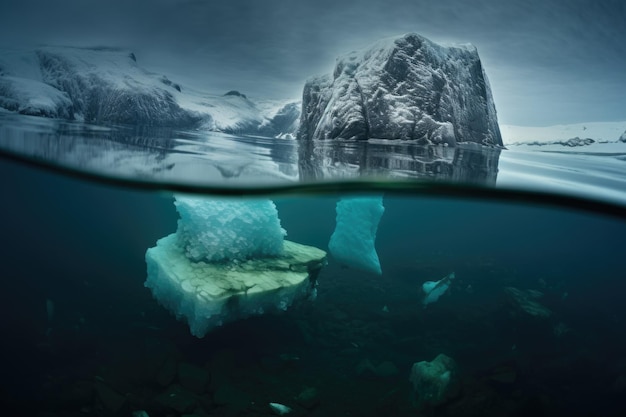This photograph captures a striking view of ice formations, spanning both above and below the waterline. The frame is split, with the lower half submerged, revealing a crystalline underwater landscape. Here, the ice showcases a palette of bright white and various shades of blue, contrasted with dark green and brown hues on the ocean floor, where a few chunks of rock and ice are also visible. The waterline itself, a swirling dark green and black boundary, divides the frame dramatically. Above the water, chunky outcroppings of ice or snow-dusted rock emerge, their surfaces tinged with black and gray. The right side of the image features a prominent outcropping, while in the background on the left, another slopes gently upwards. A strip of white snow accentuates the right background, beneath a sky heavy with mottled light and dark gray clouds. The cold, stark beauty of the icebergs and their environment is palpable, with the larger iceberg creating an almost halo effect in the distance. Scattered smaller fragments of ice float near the bottom of the frame, adding to the overall textured and layered composition.